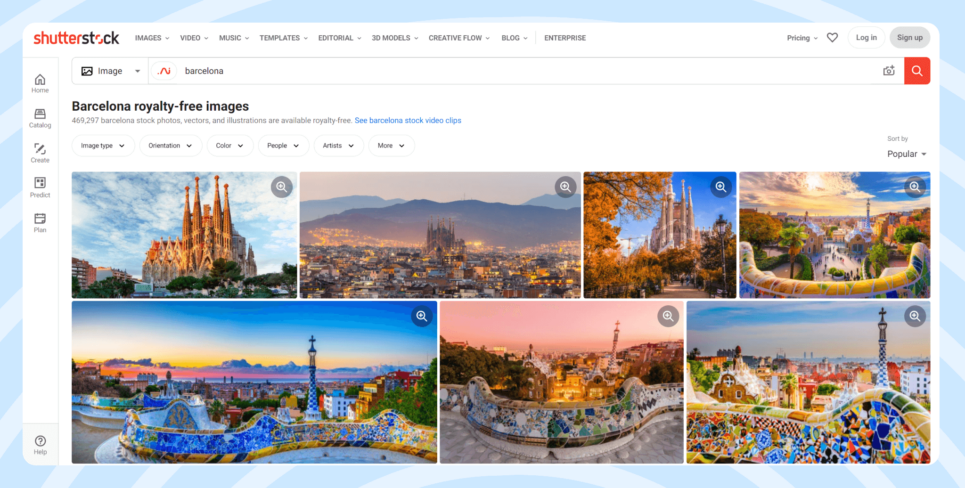The image appears to be a screenshot of a computer displaying a webpage, likely from the Shutterstock website. The background features a blue hue adorned with slanted white lines. Centered on the screen is a prominent white area. In the upper left corner, the Shutterstock logo is visible, with "Shutter" in red and "stock" in black, except the "O" which is also in red. The top of the webpage displays a menu bar with options labeled: Images, Video, Music, Templates, Editorial, 3D Models, Creative, Flow, Blog, and Enterprise. On the far right, there are links for Pricing, Log In, and Sign Up.

Centered at the top of the page is a search bar, where the word "Barcelona" has been typed. Directly beneath it, the text "Barcelona royalty-free images" is displayed in black font. Below this, there are several dropdown menus labeled: Image Type, Destination, People, and More.

In the image preview section, seven images are displayed across two rows; four on the top row and three on the bottom. The first image on the upper left features a church, set against a blue sky with clouds. The church has distinctive, elongated, slender structural elements extending from its upper portion, reminiscent of tall pipes. 

The bottom right image showcases an outdoor scene of a cityscape, highlighted by a mosaic-style wall in the foreground. The wall is composed of various colors, including blue, brown, green, and yellow, contributing to the intricate and colorful mosaic pattern.